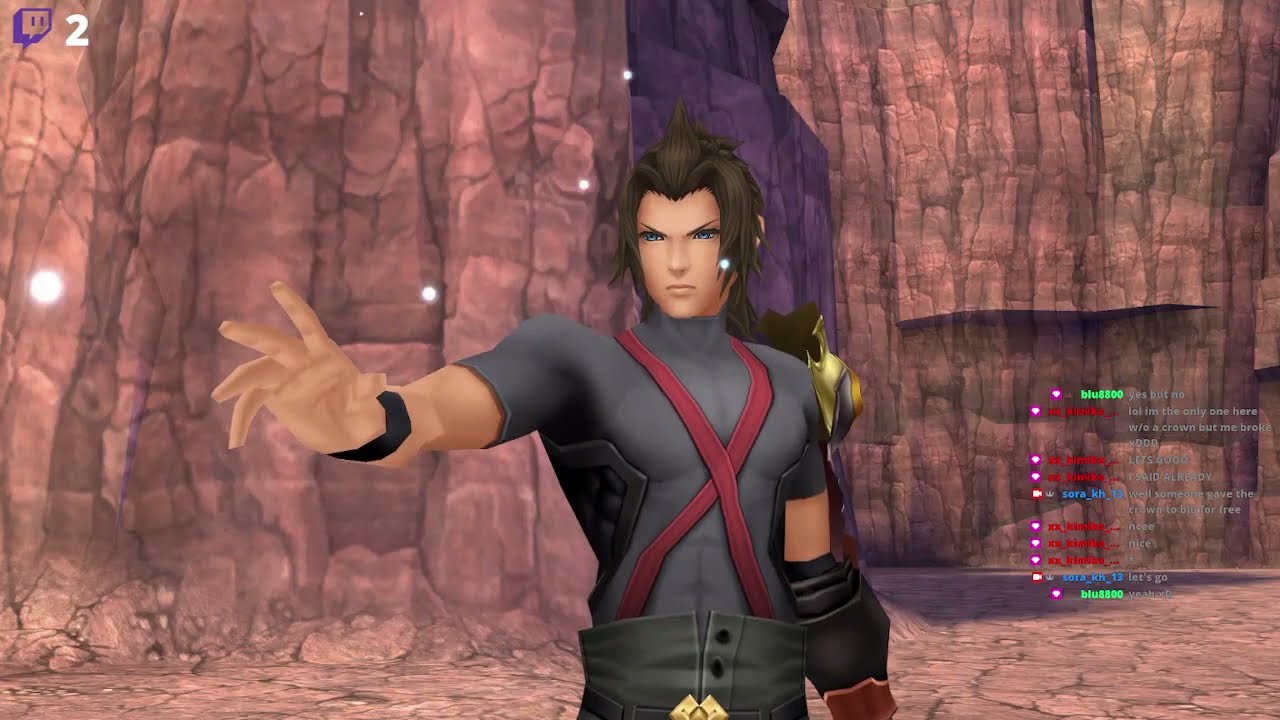The image captures a horizontal rectangular frame from a video game, specifically "Kingdom Hearts 3," featuring the character Terra. The background reveals a large, tall cliff with a brown, cracked surface, continuing down to a similarly cracked ground. The cliff's height is indeterminate as it extends beyond the top of the image. Positioned centrally is Terra, a young male character with medium-length, brown hair styled in an anime fashion. He sports a short-sleeved, dark gray shirt akin to a wetsuit, paired with waist-high buttoned pants, also gray. A gold belt buckle cinches his outfit, and red shoulder straps crisscross his torso. A hat, gold in color, dangles from his back. Terra’s right arm is outstretched towards the viewer, revealing a black wristband or watch, while his left arm, seemingly armored, hangs down out of view. On the right side of the screen is a live chat stream from Twitch, displaying various user comments in green, blue, and red text, though they are too small to distinguish clearly. The Twitch icon with the number 2 appears in the upper left corner, indicating a live broadcast. The image also contains white dots, part of the cutscene's visual effects.